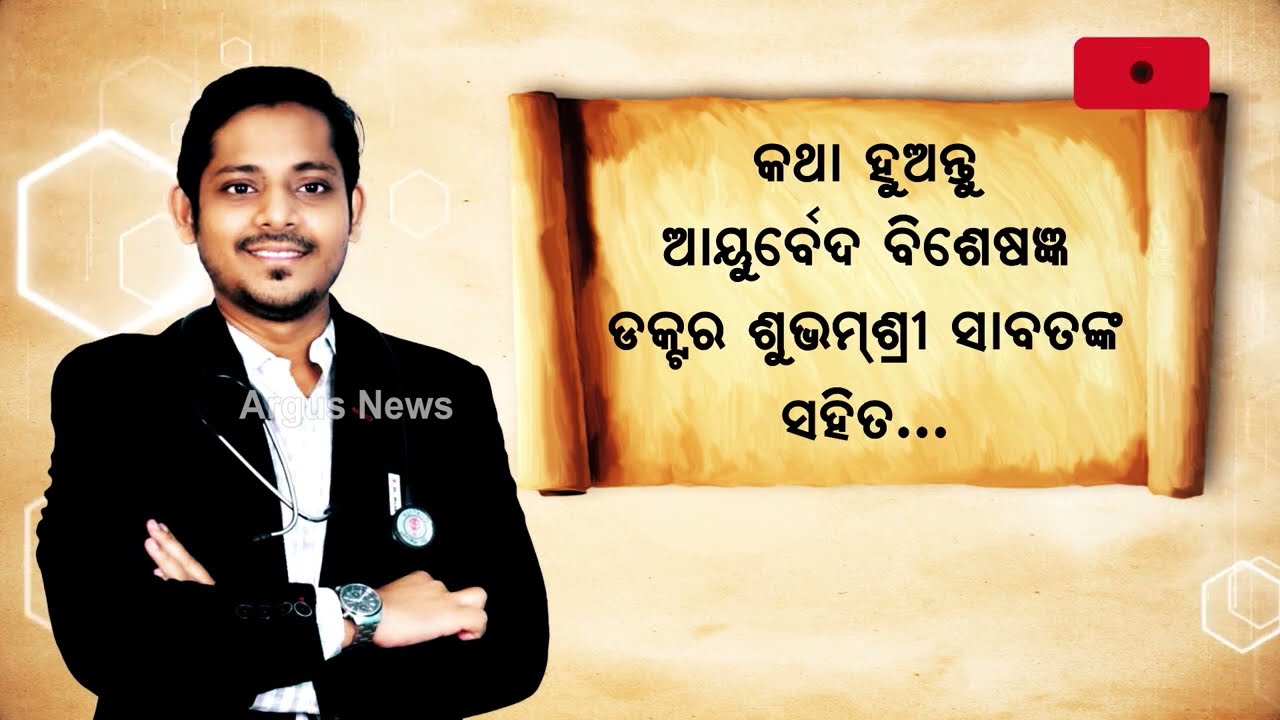The video thumbnail features a man on the left side, showing his face and upper body. He has brown skin, black hair, and a mustache coupled with a bit of beard, and is bearing a smile that reveals just his upper row of teeth. The man is dressed in a black coat over a white shirt with a collar, and he has a stethoscope around his neck, with his arms crossed in front of him. A watch adorns his right wrist. The background is a blend of various shades of beige and brown with white hexagons creating an abstract design. To the right of the man, there is a yellow scroll with text in a foreign language. At the top right corner of the image, a logo appears, consisting of a red rectangle with a black dot in its center and rounded corners. There is also a grey watermark overlaying the image that reads "Argus News."